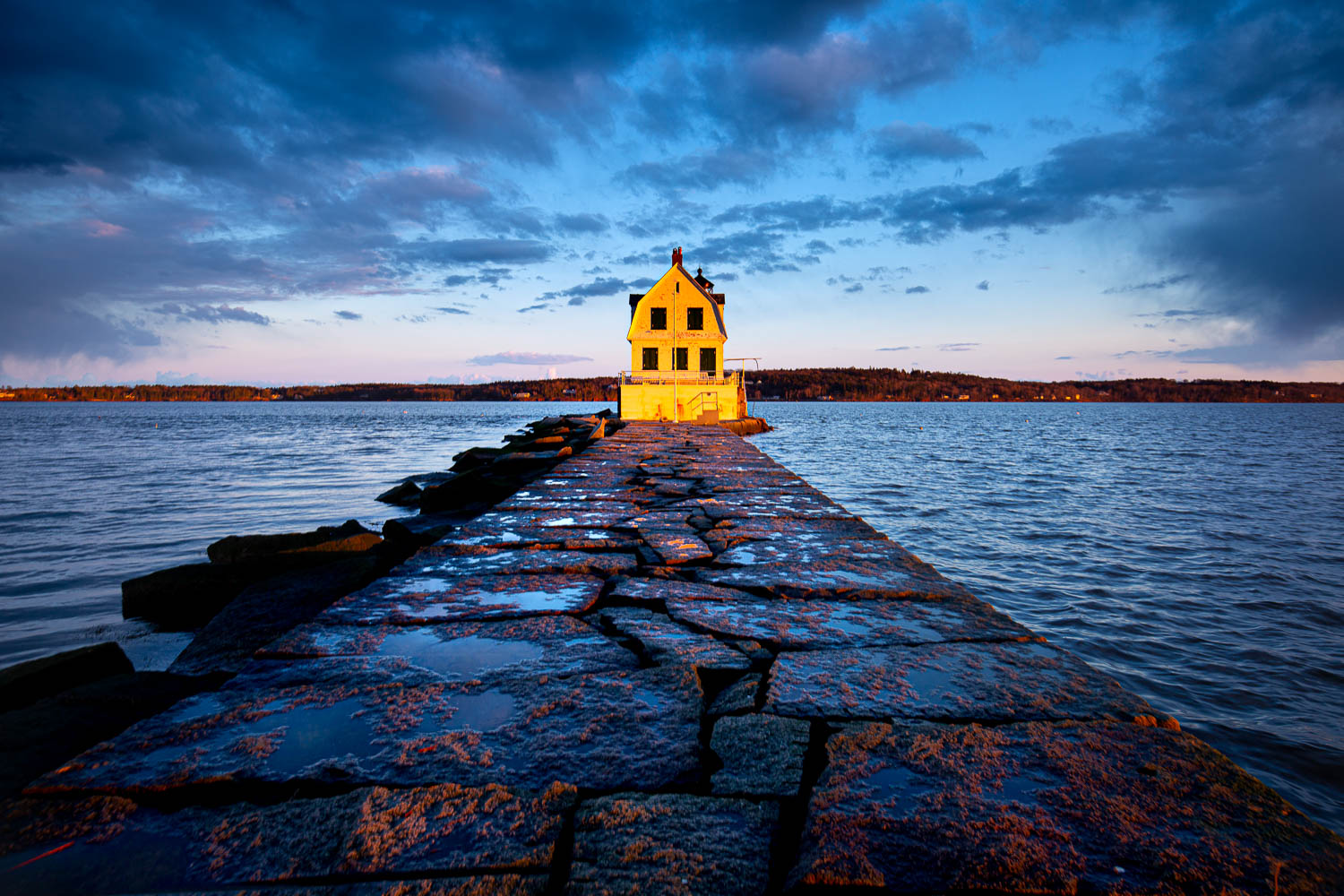At the forefront is a professionally shot image capturing an atmospheric scene at dusk. A long concrete pier or stone causeway extends roughly 100 feet into a vast body of water, potentially a lake. Flanked by large boulders and lined with some moss, the pier leads to a two-story lighthouse or possibly a boating building. The structure, which appears white or cream-colored with black shadowed windows—three on the first floor and two on the top—stands as the central focal point. The wet pier surface glistens, reflecting the moody, dark blue sky interlaced with clouds tinted purple and blue as the sun sets. Surrounding this scene is an expansive lake stretching to a distant, wooded shoreline with golden trees and rolling hills. In the background, silhouetted against the twilight, are hints of small buildings or cabins, adding depth to this dramatic and serene landscape.